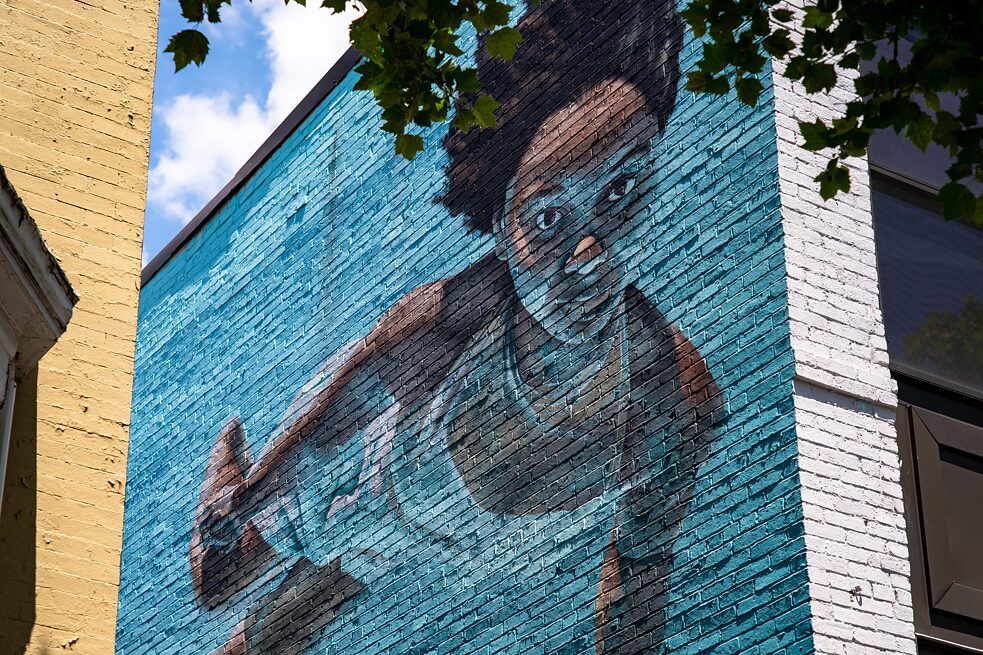The photograph showcases a vibrant mural painted on the side of a large brick building. On the left side of the image, a white-painted brick building is partially visible, adjoined by another white building partway down. Adjacent to these, the mural, set against a backdrop of blue that evokes the sense of water, features a striking depiction of an African American woman. She sports a white halter top bathing suit and a possible necklace, with her dark brown hair standing upright. The woman, who has brown eyes and a watch on her right wrist, appears to be swimming and is facing directly forward, engaging the viewer. The scene extends upward to meet the bright blue sky dotted with white clouds, and green leaves hang down from the top right, suggesting the branches of a tree. Beside the mural, past some dark glass windows and what seems to be black metal under the second window, stands another larger brown brick building. The intricate mural and surrounding elements are captured beautifully in this digital photograph.